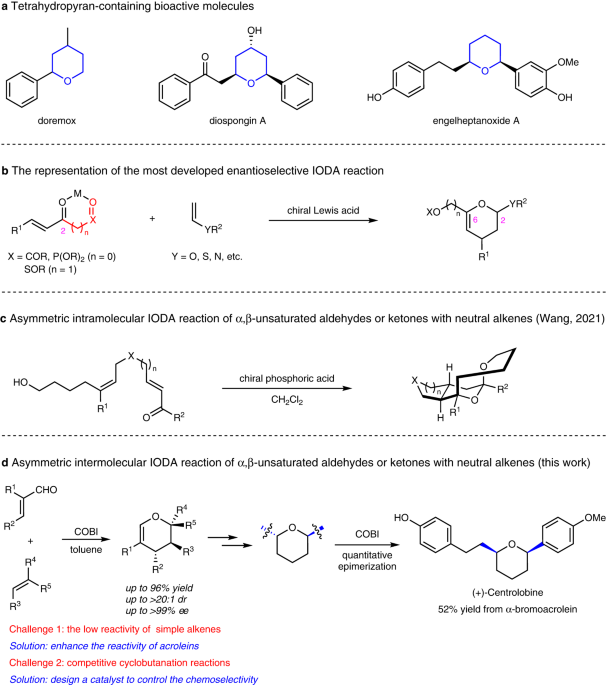This image appears to be an extract from a science textbook, likely part of a chemistry lesson. The page is divided into four distinctly labeled sections: A, B, C, and D. Section A is titled "Tetrahydropin Containing Bioactive Molecules," and it features visual diagrams of three sets of molecular structures involving hexagons and connecting lines commonly used to depict chemical bonds and compounds. Section B is labeled "Representation of the Most Developed Enantioselective Iota Reaction" and showcases three separate sets of molecular diagrams, including an arrow labeled "Chiral Lewis Acid." The other sections presumably continue the trend of displaying various intricate molecular structures and reactions. Each diagram is accompanied by descriptive text explaining the specific molecular combinations or reactions, which might be part of a multiple-choice test or an exhibit designed to challenge the reader's understanding of complex chemical processes. At the bottom of the page, colored letters indicate different challenges and solutions, reinforcing the educational purpose of the chart. The intricate details suggest that a specialized understanding in chemistry is required to fully comprehend the content.